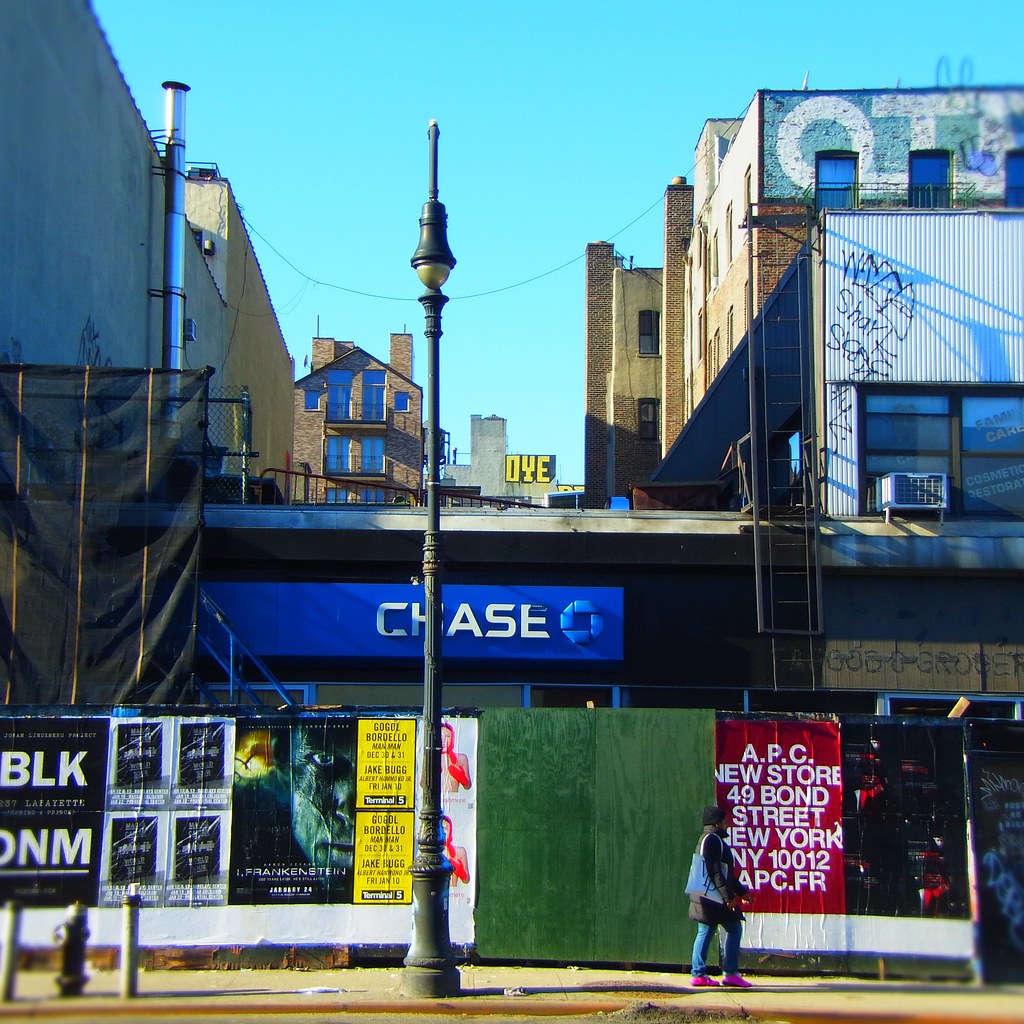This outdoor photograph captures a bustling New York City street scene with a strikingly clear blue sky overhead. Dominating the center-right of the image is a pedestrian walking from left to right, dressed in a black jacket, blue jeans, pink shoes, and carrying a blue purse. Adjacent to the sidewalk, a large streetlight stands tall, centrally positioned in the frame, while a fire hydrant sits at the far left.

The sidewalk is adorned with a variety of vibrant posters and handwritten signs attached to a makeshift wooden fence covering several storefronts. Prominently in the background, a Chase bank sign featuring the word "Chase" in white letters alongside its iconic blue logo is partially obstructed by the streetlight. Nearby, another storefront displays a red sign with white lettering that reads "APC new store, 49 Bond Street, New York, New York 10012."

Further back in the scene, a second-story building sports graffiti, adding to the urban aesthetic. Brick buildings rise in the distance, completing the cityscape, which is bathed in the natural light of the day. The image encapsulates the vibrant energy and layered visuals of a typical New York City street.